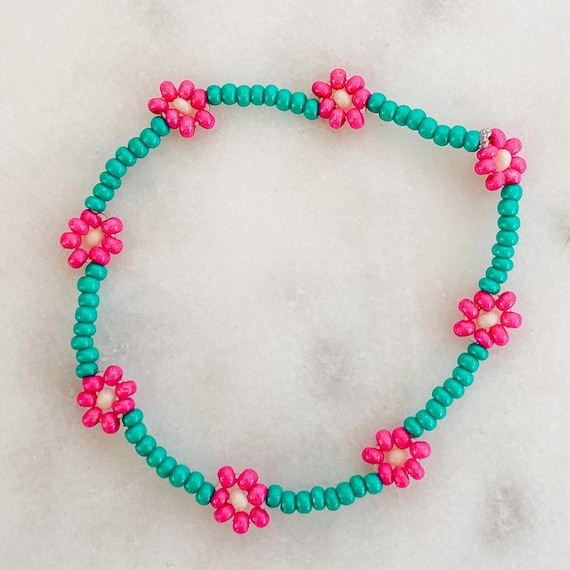This close-up image showcases a beaded jewelry piece, likely a bracelet given its intricate size and detailing. The bracelet features a series of charming flower motifs and beads, arranged in an eye-catching pattern. Each flower is made up of seven pink petals with a creamy white center. These floral sections are separated by stretches of eight turquoise beads, creating a vibrant and festive design reminiscent of a Hawaiian lei. There are eight floral sections in total, with each turquoise length consistently comprising eight beads. The entire piece rests on a semi-translucent white or beige surface, probably tissue paper, which serves as the simple yet effective background, highlighting the bright and beautiful colors of the bracelet. The photograph is rectangular, focusing closely on the detailed craftsmanship of the piece.